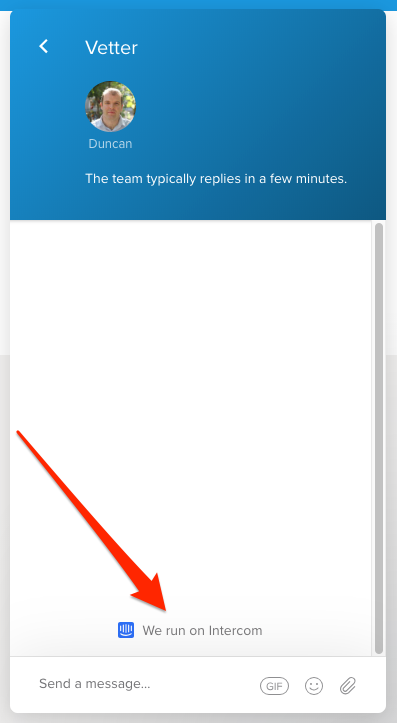This image is a screenshot of a smartphone interface. It features a gray border on the left, right, and bottom edges. The background of the screen is predominantly white. At the top, there is a thick section with a gradient color transition from light blue to dark blue. Within this section, there is a circular profile picture of a person named Duncan, who is looking directly at the camera.

Above Duncan's image, the text "VETTER" is displayed in capital letters, alongside an arrow pointing to the left. Below Duncan's picture, there is a message in white text stating, "The team typically replies in a few minutes."

The lower section of the image is also white. There is a red arrow originating from the center left side of this section, pointing towards text that reads, "We run on Intercom." To the left of this text, there is a blue square icon with white lines.

At the very bottom of the image, in thin gray font, it says "Send a message." To the right of this text, located at the bottom right corner, are three icons: a GIF icon (labeled "GIF"), a smiley face for emojis, and a paperclip icon for attachments.